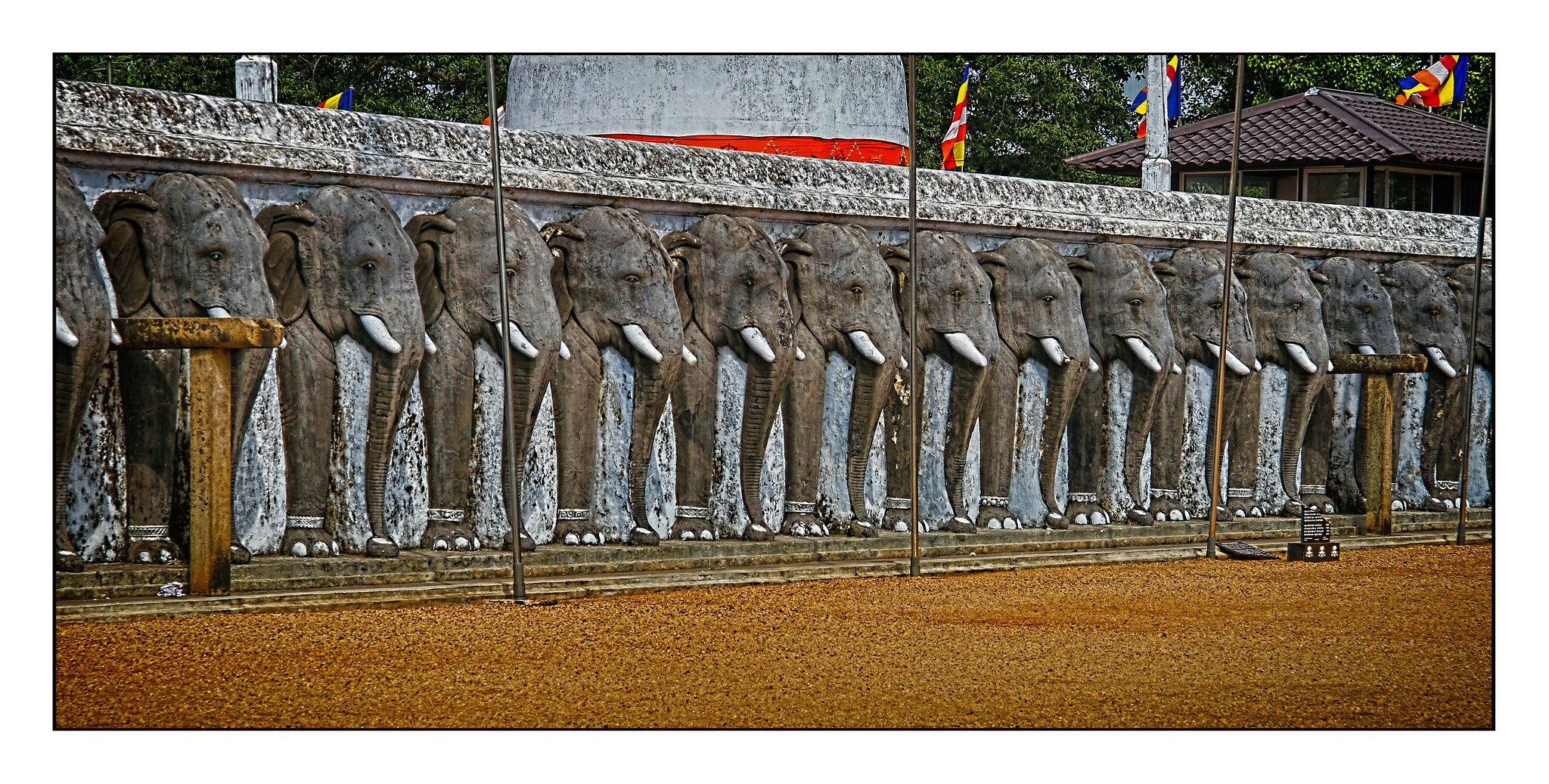This photo shows a detailed scene seemingly taken in a foreign country, featuring a prominent stone wall adorned with intricate elephant carvings. The elephants, approximately 15 in number, are 3D reliefs in a grayish-brown tone with white tusks, and each features one visible leg with black decorative shackles and discernible toenails. Extending from the left corner to the right, the wall is highlighted by a gray stone border and stands on a light brown, possibly dirt, ground. Above the wall, there are various flags in red, white, yellow, and blue, though their significance is unclear. In the background, a building with ornate roof tiles and a red and white column tower behind it adds to the scene's exotic ambiance.